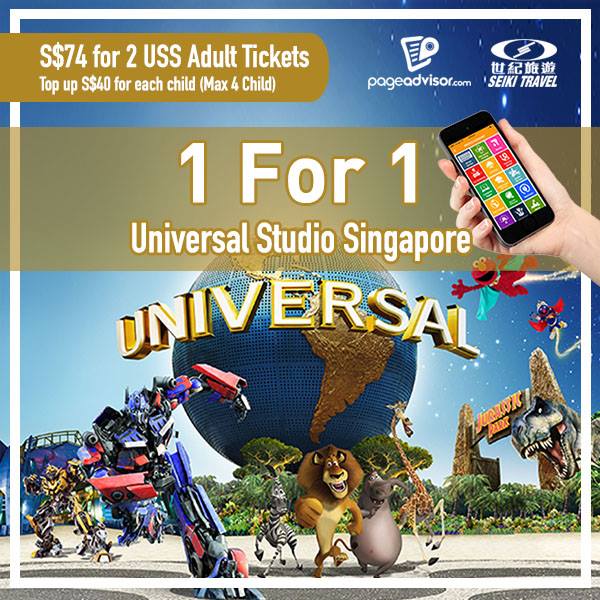The image is a vibrant and detailed screenshot of an advertisement for Universal Studios Singapore. Dominating the background is a large blue globe with gold-colored continents, the emblematic centerpiece of Universal Studios. Prominently wrapped around the globe is the word "Universal" in bold white letters outlined with gold. 

On the sidewalk in front of the globe, various beloved characters are vividly showcased. Two towering Transformers stand guard, exuding an aura of strength and excitement. Next to them, characters from the animated movie Madagascar add a playful touch with a zebra, a lion, a hippo, and a giraffe appearing life-like and cheerful. An iconic Jurassic Park arch looms in the scene, featuring a lifelike, menacing T-Rex with its jaws wide open, seemingly prowling from the right side of the image. Adding a whimsical note, Elmo energetically flies through the air, donning a light blue cape.

A person's hand, appearing on the right side of the photo, brandishes a smartphone, suggesting the accessibility and modern convenience of booking tickets.

The promotional text at the top declares a special offer: "Singapore $74 for two USS adult tickets. Top up S40 for each child, max four a child." Further information directs viewers to PageAdvisor.com and Seiki Travel (spelled out as S-E-I-K-I), indicating the source and partnership for this remarkable offer.

The image distinctly avoids showing any real people, animals, or airplanes, focusing solely on the immersive attractions and the promotional details.

This captivating advertisement effectively communicates the excitement and adventure that awaits visitors at Universal Studios Singapore.